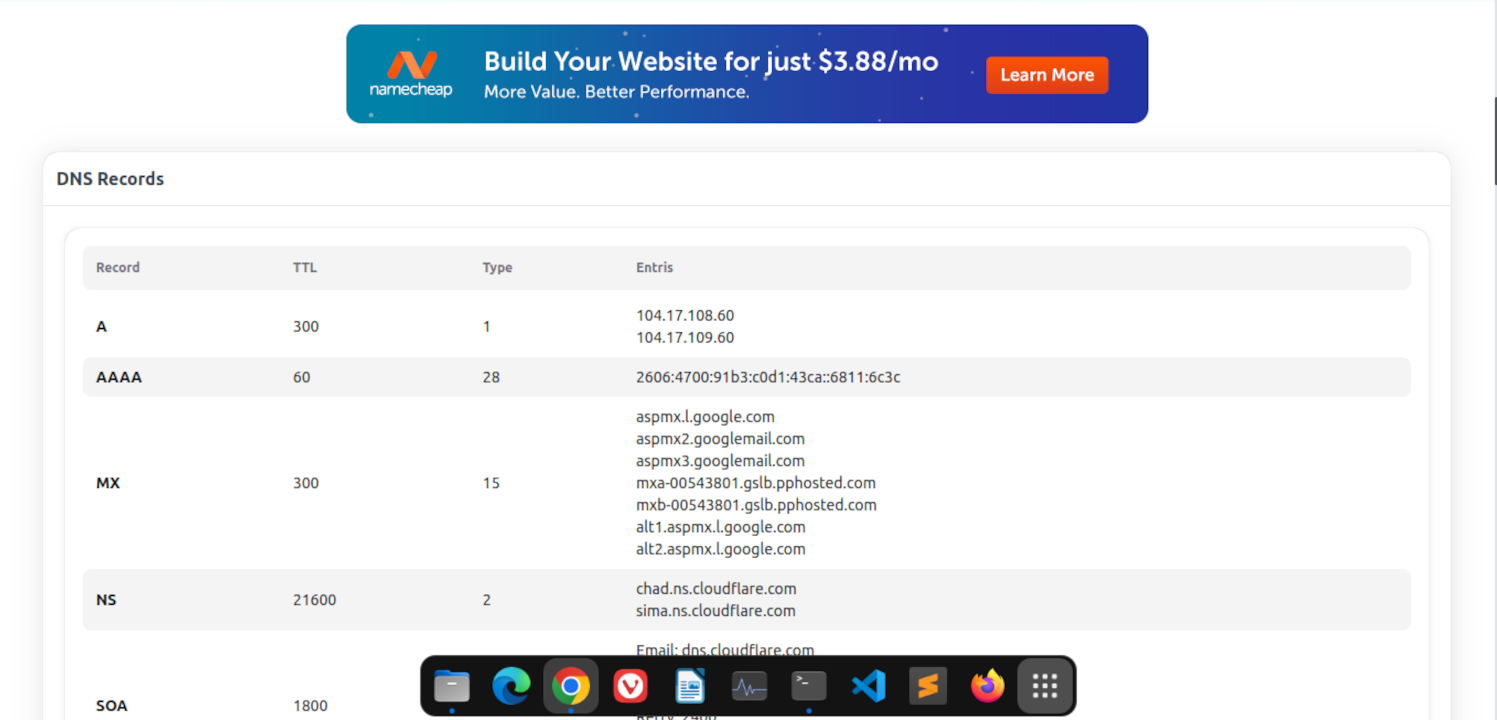This image showcases a detailed webpage view, starting with an advertisement at the top. The ad, promoting Namecheap, boasts a slogan "Build your website for just $3.88 a month - more value, better performance." Below this, an orange "Learn More" button is set against a vibrant blue background adorned with assorted colors, attracting user attention.

Beneath the ad, the focus shifts to the DNS records, where a section titled "Records" displays a series of icons and numbers. The records include:
1. Type A with a TTL (Time to Live) of 300.
2. Type AAAA with a TTL of 60.
3. Type MX with a TTL of 300.
4. Type NS with a TTL of 21,600.
5. Type SOA with a TTL of 1,800.

Each record type is paired with specific numerical identifications: Type A (1), Type AAAA (28), Type MX (15), and Type NS (2). Additionally, the page is interspersed with various emails and other numbers indicative of DNS configurations.

At the bottom of the page, a dock bar features a collection of icons representing different applications and browsers. This includes a file holder icon, the Edge browser icon, Google Chrome, Firefox, and several other program icons typical of those found on a laptop or desktop computer.